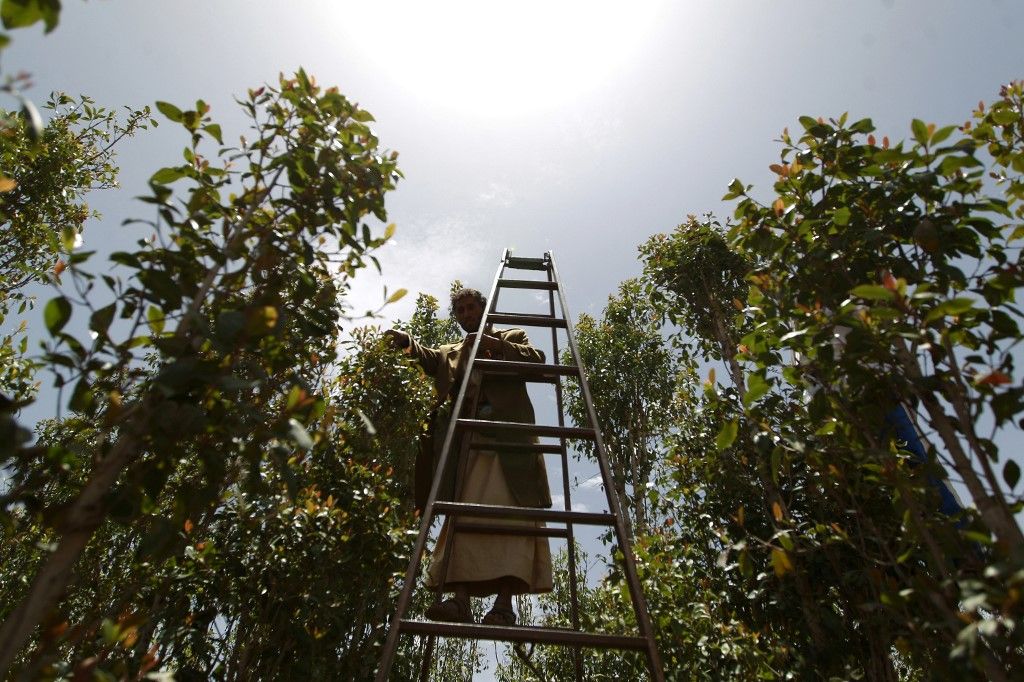The photograph captures a dramatic worm's eye view of an orchard bathed in intense sunlight. At the center of the image is a large double folding ladder, reaching towards the sky. A person, possibly a man, is positioned midway up the ladder. Although the person's features are indiscernible due to the blinding, overhead sun, their attire—comprised of a long beige dress-like garment and a coat (or tunic and blazer)—suggests they may be from the Middle East or Southeast Asia. The orchard is filled with tall, narrow, healthy trees bearing indistinct fruit, which could be dates, lemons, or perhaps pears. The sky above is a muted gray, with sunlight piercing through the clouds, casting sharp contrasts of shadows and highlights across the scene. In the person's hand is an object that might be a device, possibly used for taking pictures or for harvesting the fruit. The entire composition evokes the hard work and serenity of fruit picking against the backdrop of a bright, possibly midday sun.